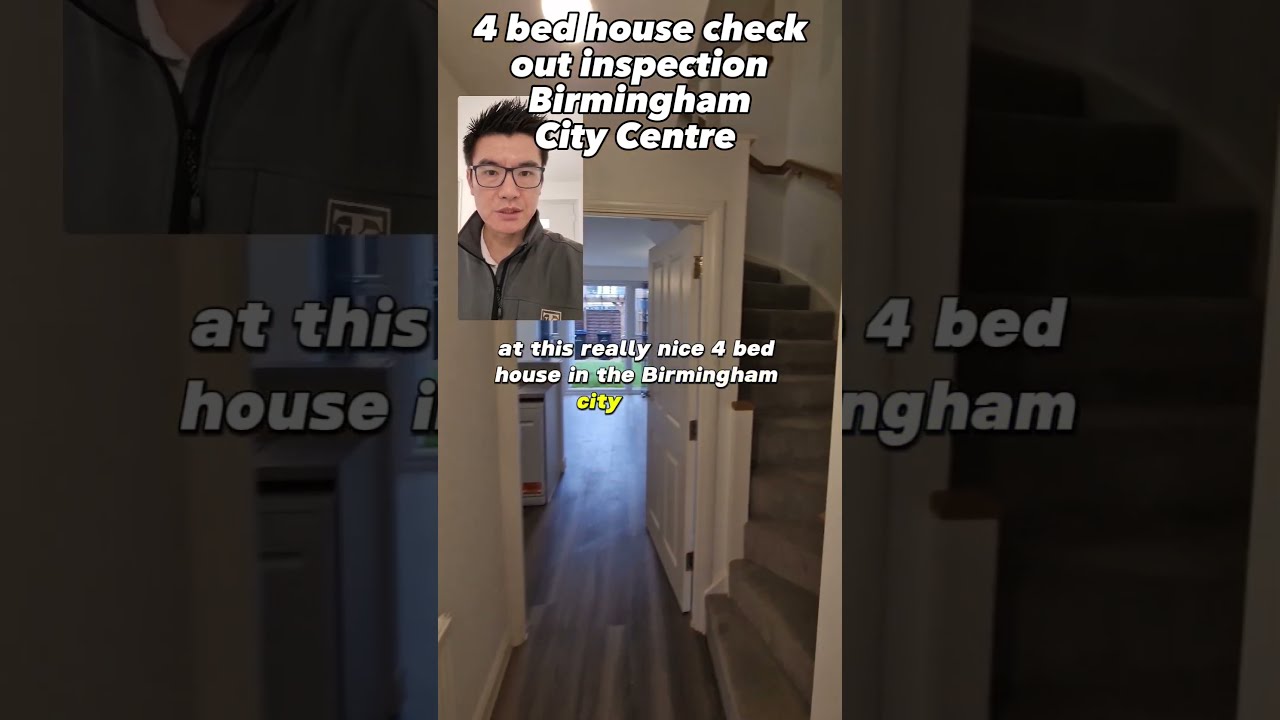This detailed vertical cell phone image portrays the entryway of a home, marked by polished hardwood floors, white walls, and a doorframe that opens up into what appears to be a kitchen area. Immediately visible are stairs to the right, leading to the upper floor, and a sliding glass window that looks out into a backyard featuring a garbage can and a recycling bin. At the top of the image, bold white text reads "Four Bed House Check Out Inspection, Birmingham City Centre," with a smaller font mid-image stating "at this really nice four bed house in the Birmingham City," where the word "City" is highlighted in yellow. Interspersed within these text captions is the image of an Asian man with short black hair, wearing glasses and a brown jacket, seemingly in the middle of speaking, possibly showcasing the house for an online inspection or sales pitch.